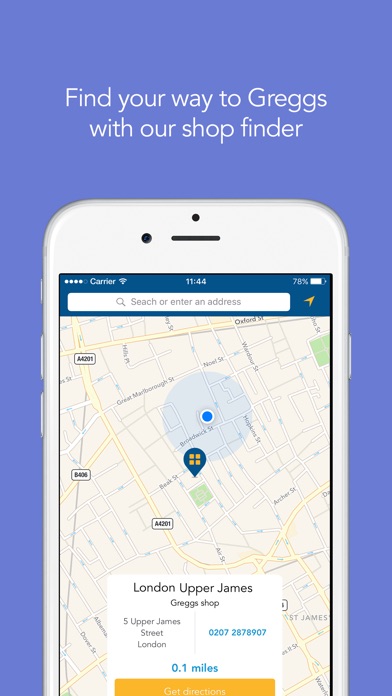The image showcases an advertisement for a smartphone application, specifically designed to help users locate Greggs shop locations. The top portion of the image features a blue gradient background with white text that reads, "Find your way to Greggs with our shop finder." The central focus is on a white smartphone displaying the app's interface.

The smartphone screen prominently displays a stylized map with yellow and blue lines representing major roads and intersecting streets. A blue dot with a surrounding radius circle represents the user's current location, slightly above and to the right of the center, resembling an epicenter. Additionally, four small yellow squares and a blue pin indicate key points on the map.

Towards the bottom of the smartphone screen, there is a white dialog box containing detailed information about a Greggs shop. The text includes the location marker "London, Upper James," followed by the address: "5 Upper James Street, London." Below the address, a numerical series that likely represents geographical coordinates is displayed, along with the distance "0.1 miles" in blue text. The "Get Directions" button is highlighted in orange with white lettering, providing a call-to-action for users.

The advertisement skillfully combines visual elements and essential information to illustrate the app's functionality and ease of use in finding the nearest Greggs shop.